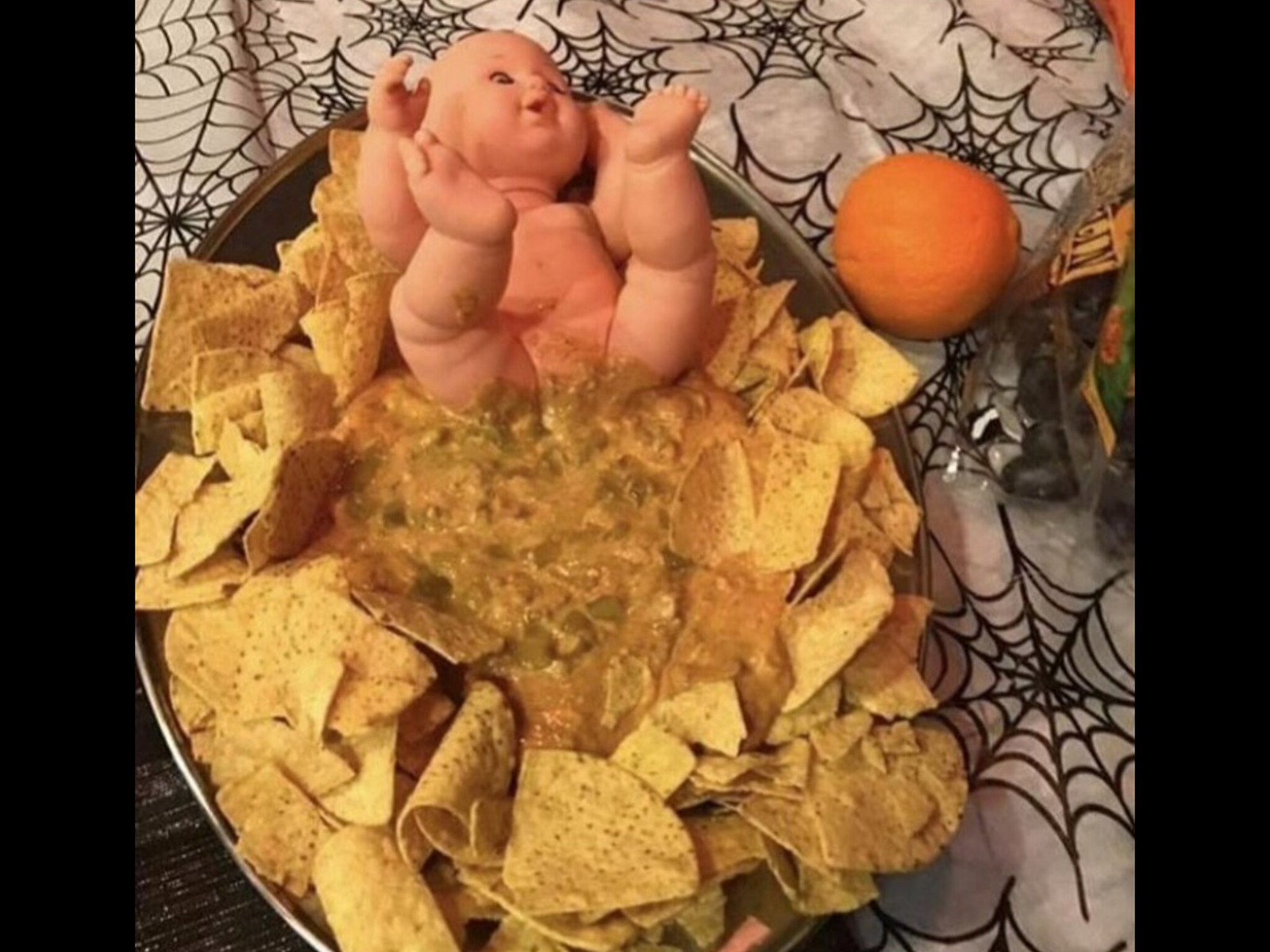This image features a humorous and slightly vulgar Halloween display set on a table adorned with a white plastic tablecloth decorated with cobweb patterns. At the center is a large oval silver bowl filled with a bed of tortilla chips surrounding a mix of greenish cheese and refried beans dip. A naked plastic baby doll is placed in the middle of the dip, positioned with its arms and legs up, mimicking the appearance of a baby having a diarrhea accident all over the chips. This quirky setup is further accented by an orange and possibly a package of candy or party favors placed next to it on the table, enhancing the holiday theme.